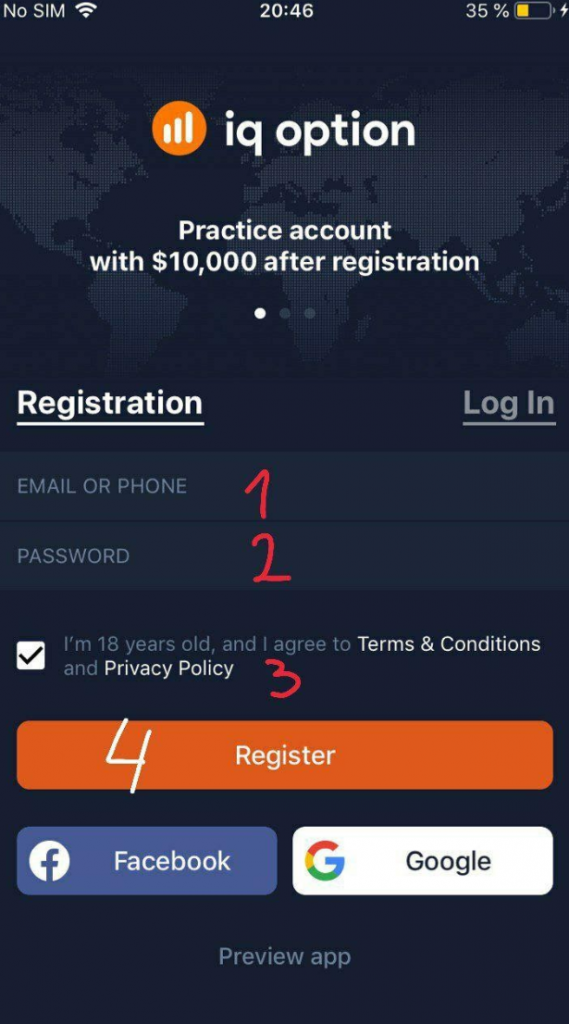Caption: 

The image displays the homepage of the IQ Option website, prominently featuring a sign-up form for a practice account. Users are prompted to enter their email or phone number, create a password, and agree to the terms before registering. The background showcases a world map, lending an international feel to the site. The design is clean and straightforward, suggesting an intuitive user experience for those interested in IQ tests or related activities.